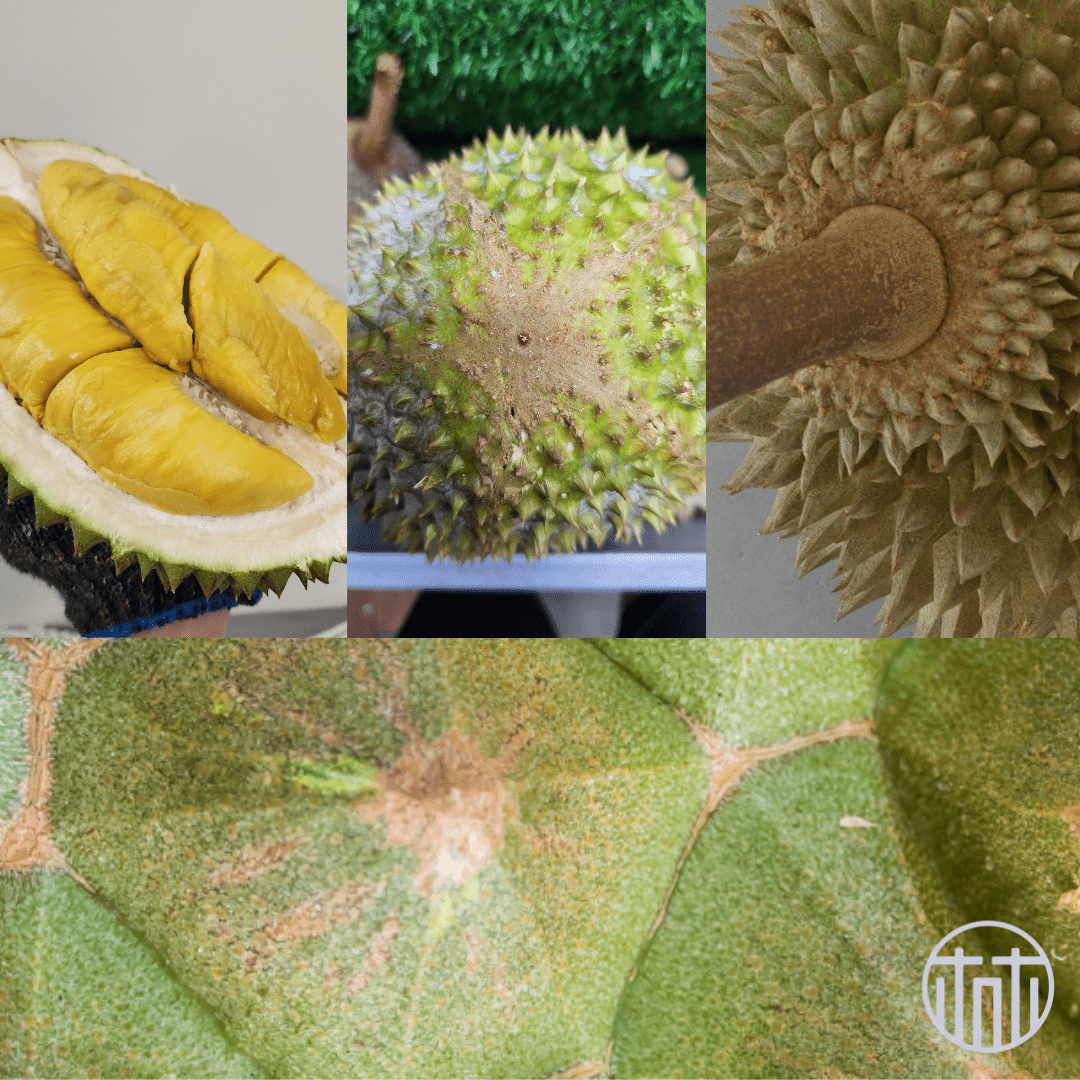The image is a collage consisting of four photographs depicting a peculiar fruit or vegetable in various stages and perspectives. The top row features three photos. Starting on the left, the first image showcases a yellow-centered fruit with a green, spiky exterior and a white base, held by a person wearing a gray glove. The central photo illustrates the same fruit turned over, revealing green spikes radiating from a brown star-shaped core, with green foliage in the background. The rightmost photo presents a close-up of the fruit on a brown stalk, with green protrusions tinged with light brown, resembling the underside of a green sunflower. The single photograph on the bottom spans the width of the collage and displays large, overlapping, circular green leaves with brown centers, akin to lily pads.